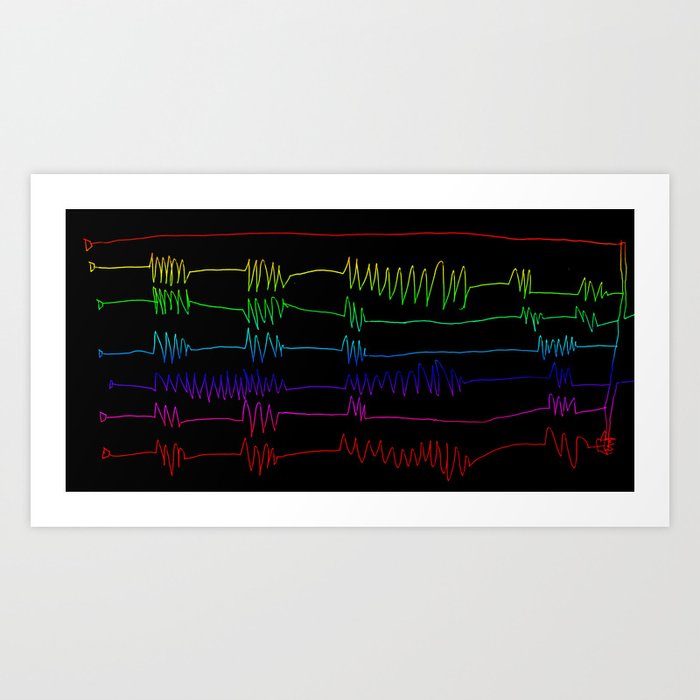The image features a detailed drawing resembling a heartbeat monitor display against a black background, bordered in white with a surrounding light blue backdrop. Across the central black area, various colored lines run horizontally from left to right, each depicting unique waveforms. At the very top, the red line emerges from a letter 'D' on the left and progresses straight to the right. Below, a yellow line also starts from a 'D' and displays a waveform pattern. Subsequent lines include green, light blue, dark blue, purple, and another red, each presenting different degrees of squiggles and movements. The lines are not parallel, creating a dynamic and varied graphical representation.